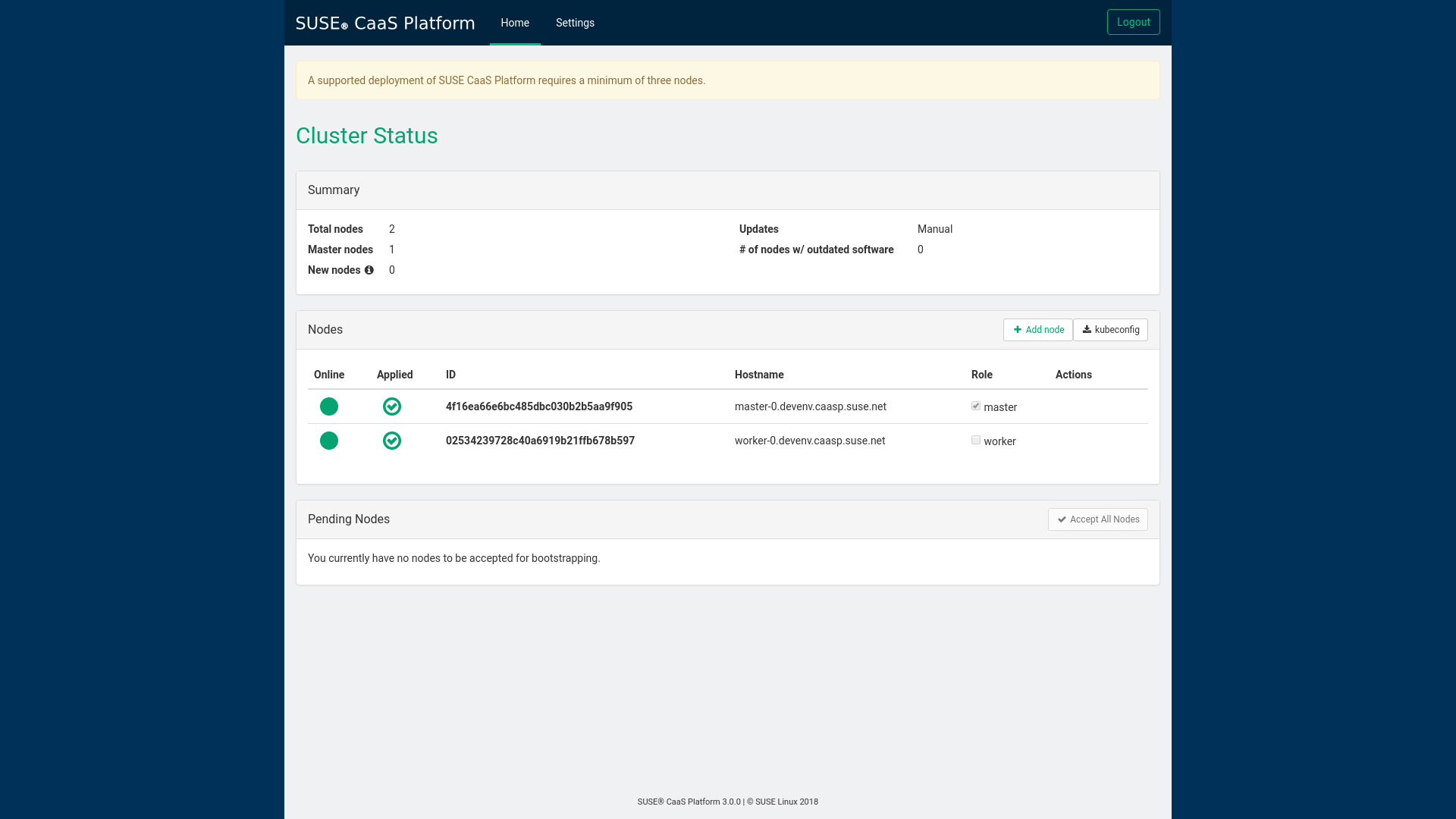The image depicts a detailed web page interface for the SUSE CaaS (Container as a Service) Platform, set against a dark blue background with white text. At the top of the page, the SUSE logo is prominently displayed alongside the sections labeled "CaaS Platform," "Home," and "Settings."

Below these headers, there is a light pink notification box that states: "A supported deployment of SUSE CaaS Platform requires a minimum of three nodes." Directly under this notification, the "Cluster Status Summary" is presented, summarizing the system's current state:

- **Total Nodes:** 2 
- **Updates:** Manual

Further down, detailed information about the nodes is provided:

- **Master Nodes:** 1
- **Number of nodes with outdated software:** 0
- **New Nodes:** 0

Following this summary, a white rectangular box lists the nodes that are online. The headings within the box read: "Nodes Online," "Applied ID," "Hostname," "Rule," and "Actions." The current entries are as follows:

1. **Master Node:**
   - Status Indicator: Green button
   - Status Check: Checkmark icon
   - Node Details: Alphanumeric ID
   - Hostname: master-0.Devalx.ksap.suse.net
   - Rule: Master

2. **Worker Node:**
   - Status Indicator: Green button
   - Status Check: Checkmark icon
   - Node Details: Alphanumeric ID
   - Hostname: worker-0.devalx.ksap.suse.net
   - Rule: Worker

Lastly, the section labeled "Pending Nodes" indicates: "You currently have no nodes to be accepted for bootstrapping."